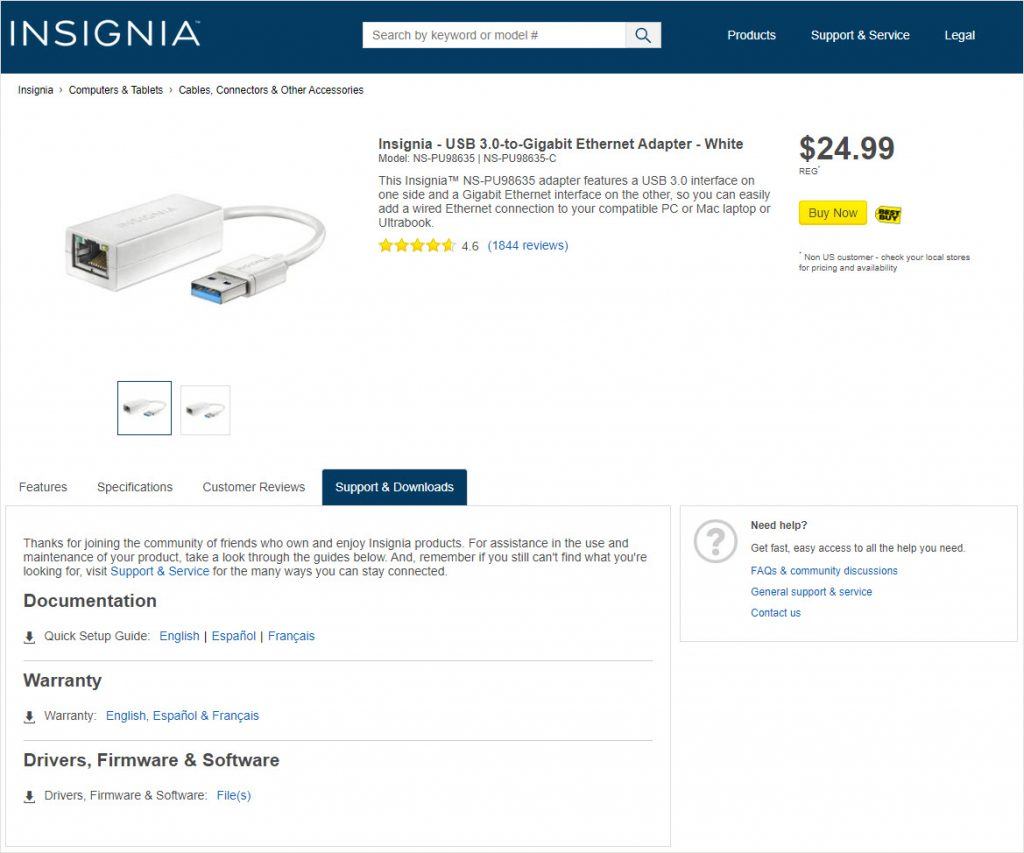This is a detailed description of a product page from either Best Buy or a similar website, accessed via a desktop or laptop computer. The header is a dark navy blue, featuring the brand name "INSIGNIA" in large, white, capitalized letters on the left side. Centrally located in the header is a search bar with the placeholder text "Search by keyword or model number." To the right of the search bar, there's a menu with options such as "Products," "Support & Service," and "Legal," all in white font.

The main content area showcases the product being viewed. On the left side, there is a main photo of the product with two smaller clickable thumbnails below it, displaying alternate views. To the right of the images is the product's title: "Insignia USB 3.0 2 Gigabyte Ethernet Adapter - White," accompanied by a concise four-line product description.

Below the product title and description, there are customer ratings indicated by yellow stars. It shows a rating of 4.6 accompanied by 1,844 reviews, clickable via blue text. The price of the product, $24.99, is prominently displayed next to a yellow "Buy Now" button with the Best Buy logo beside it.

Towards the bottom of the page, there is additional information, which includes documentation such as the setup guide, warranty details, and firmware/software updates. The page is well-organized and provides all essential details for a potential buyer.